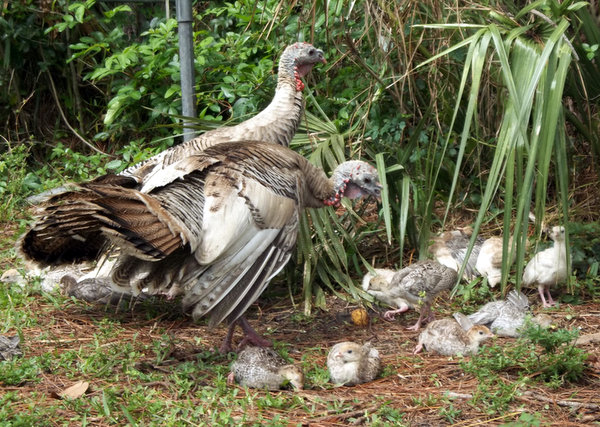In this detailed landscape photograph of an outdoor scene, a family of turkeys is prominently featured. The foreground showcases two large adult turkeys, identifiable by their long necks and the red coloration under their beaks. Their plumage includes a mix of predominantly white with brown accents on their tails and some black markings. The coloration varies between gray, white, and beige shades. Accompanying them are at least eight recently hatched baby turkeys with gray and white down, dispersed on the grassy terrain. The adult turkey on the left, appearing protective, looks down at the chicks, which are engaged in various activities such as pecking and grazing.

The backdrop includes a mixture of verdant greenery and shrubs, with some portions exhibiting dead brown grass. In the top right corner, long strands of grassy plants and other foliage are visible, adding depth to the scene. The overall setting appears to be a transitional area between open grassland and denser foliage, suggesting a natural, perhaps forested environment where birds and plants coexist.